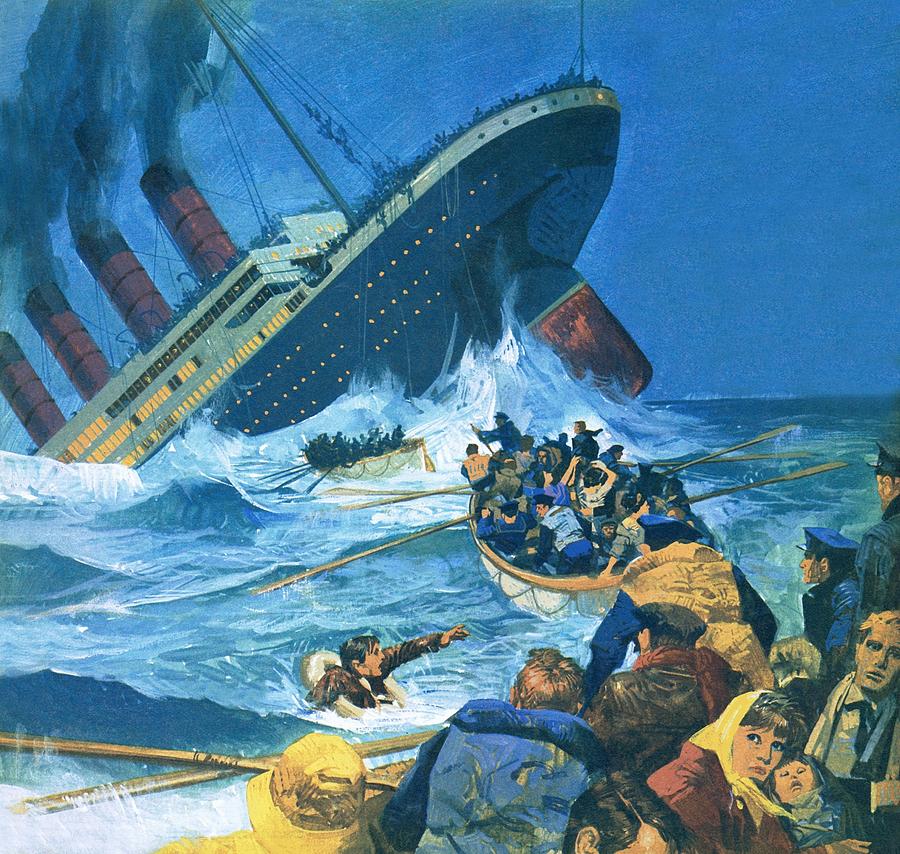This detailed illustration captures the tragic sinking of the RMS Titanic. Dominating the upper left part of the image, the mighty vessel's bow is already submerged, while its stern rises high out of the water, exposing the massive propellers. The Titanic's smokestacks, distinctly red at the base and black at the top, belch dark smoke despite the ship's dire state. Below the stacks are several white decks still aglow with lights, contrasting sharply with the dark blue of the doomed North Atlantic night. The hull shows rows of illuminated windows, a futile warmth against the frigid waters lapping higher with each passing moment.

In the lower right portion of the image, a lifeboat filled with desperate survivors rows away from the sinking leviathan. Among them, a woman in a yellow kerchief clutches a baby close, while a man in a blue vest stares back at the Titanic, the gravity of the disaster etched on his face. Beside the lifeboat, a person in a brown suit floats in the icy sea, clinging to life with a life vest. Two engineers, likely from the ship itself, stand in the lifeboat, their expressions somber as they witness the end of an era.

In the chaotic scene around the ship, other lifeboats are visible, filled with more survivors rowing frantically to escape the impending danger of being pulled under by the ship's suction or overturned by the turbulent waters. The night sky is a deep, foreboding blue, mirroring the harrowing plight of the passengers.

This artwork, while dramatic, takes some artistic liberties. It inaccurately shows steam still emitting from the Titanic’s smokestacks and lights brightly shining, elements that would not have persisted once the lower compartments were flooded and the engines ceased to function. Nevertheless, the image powerfully encapsulates the fear, desperation, and tragedy of one of history's most infamous maritime disasters.